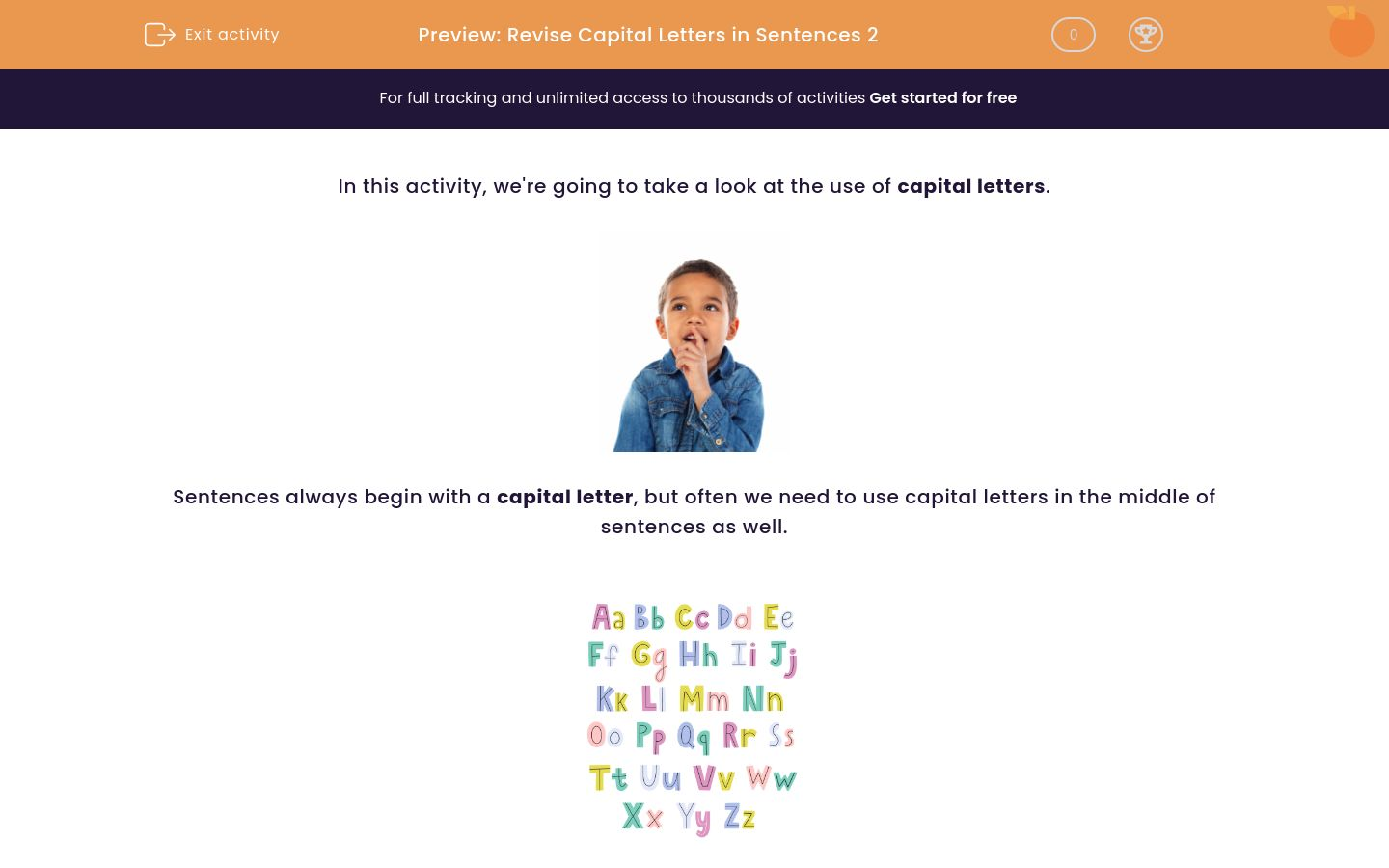This is a screenshot of an educational website designed for young learners. The main background of the site is white, prominently featuring a small boy in a blue jean jacket at the center. The boy appears to be in the midst of telling a story, with his finger raised to his mouth. Below this image, a significant text is displayed: "Sentences always begin with a capital letter, but often we need to use capital letters in the middle of sentences as well." 

Beneath this instructional message, the entire alphabet is presented in both capital and lowercase forms. The letters are colorful, ranging from reds, pinks, greens, blues, purples, to yellows, much like you would see in educational materials aimed at preschool to early elementary school students. The alphabet is arranged in a clear, structured format with the letters starting from A at the top and ending with Z at the bottom, creating a visually engaging collage-like display.

At the very top of the webpage is an orange banner. In the center of this banner, a title reads: "Preview Revised Capital Letters in Sentence 2." This header further hints at the educational content aimed at teaching proper capitalization within sentences.